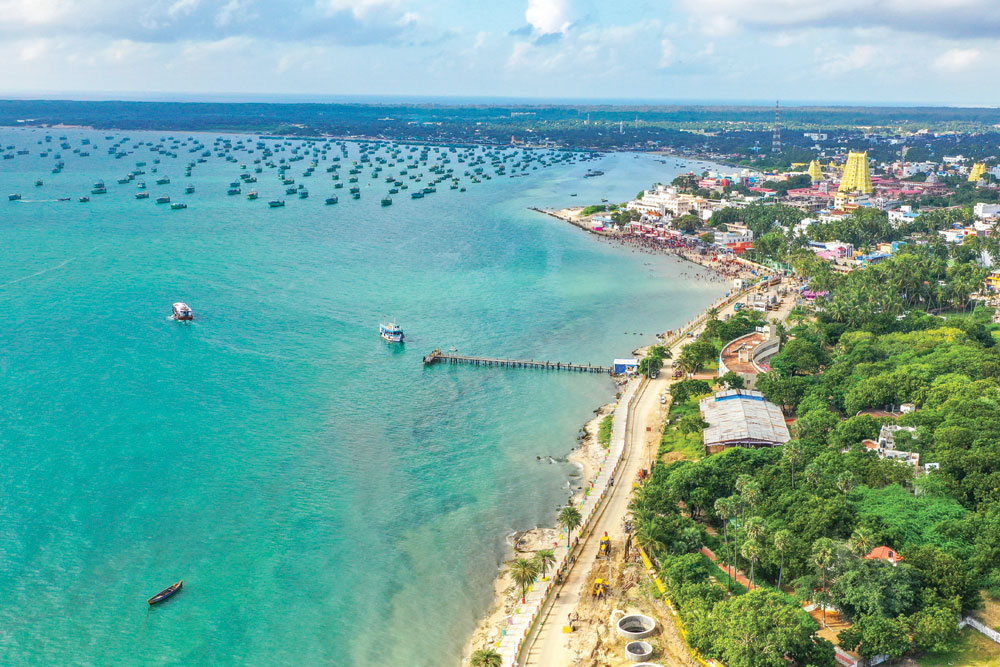This is a detailed aerial photograph taken in daylight, showcasing a picturesque coastal scene. The majority of the image is dominated by the bluish-green ocean, which occupies the left side. The shoreline starts from the lower portion of the frame, stretching diagonally upwards to the right. To the right of the shoreline, there's a narrow, sandy beach, bordered by lush green grass and trees.

In the upper left background, a variety of boats dot the water, including a small rowboat and two larger vessels. Closer to the coast, a pier juts out into the water. The upper right background reveals a city skyline in the distance with tall buildings, including a prominent large yellow building and a tower. There’s also a building closer to the shoreline in the foreground.

The sky is a bright blue, adorned with fluffy white clouds that extend across the top of the photo. Along the shore, a walking path meanders parallel to the coastline. Overall, the image captures the serene beauty of the coastline, the busy activity of boats on the water, and the distant hint of an urban landscape under a clear, sunny sky.